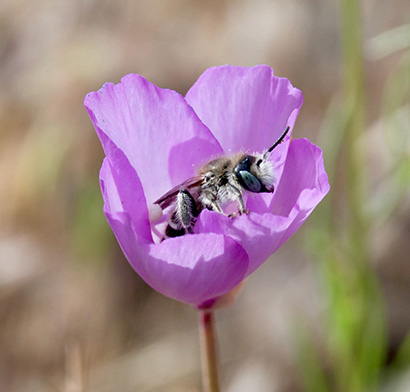The image showcases a close-up of a deep lavender-purple flower, possibly a rose, with a beige-brown base. The foreground prominently features this flower, while the background is softly blurred, revealing hints of green buds sprouting and a stem. Centered in the flower are two bees: one on the left and one on the right, actively pollinating and feeding on the flower. One bee, covered in a bit of fur and primarily black with some white on its upper head, is visibly crawling within the petals. The insect's characteristics, such as its large eyes, black antennas, and blue-tinted eye, are clearly noticeable in the detailed shot. The overall setting appears to be outdoors, capturing the essence of nature with an emphasis on the intricate interaction between the bees and the vibrant flower.